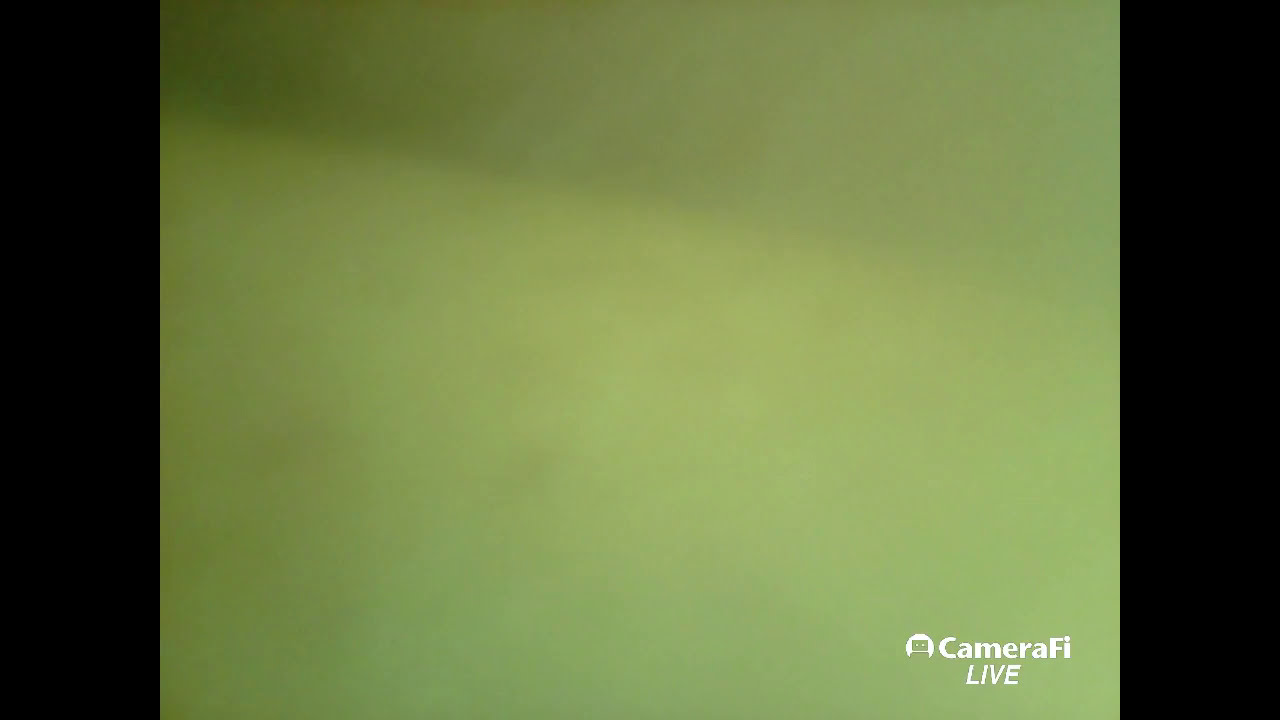The image is a rectangular picture with a solid green square at its center. The top and bottom sides of the rectangle are twice as long as the left and right sides. The green square in the center transitions from a darker green at the top to a regular green in the middle, and finally a lighter green at the bottom. The image is framed on both the left and right sides by vertical black bars running from top to bottom. In the bottom right corner of the green section, there is white text that reads "CameraFi Live," with "CameraFi" spelled C-A-M-E-R-A-F-I and "Live" spelled L-I-V-E. To the left of this text, there's a logo resembling a white, upside-down "U" with two dots and a line inside, suggesting eyes and a mouth or headlights in a garage-like structure.